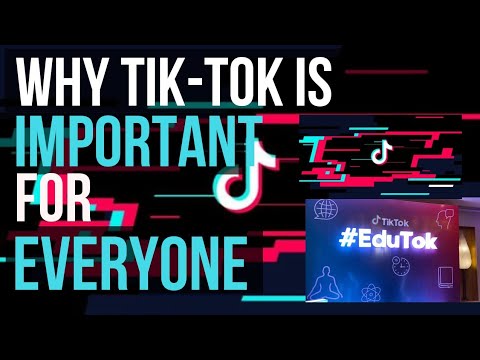The image features an advertisement-like header against a black background with a digital effect reminiscent of TV scan lines and a pixelated aesthetic. The background showcases vibrant hues of blue and reddish-pink. Positioned on the right side is the TikTok logo, while a larger TikTok logo is prominently placed at the center. Overlaid text in white reads, "Why TikTok is Important for Everyone," with "why" and "for" in blue, and the rest in white.

In addition, there are screen captures of the TikTok background, featuring the centered TikTok logo. The backdrop also includes a wall decoration for an event, with the text "TikTok #EduTalk" displayed in white against a blue and purple gradient background. The decor appears to belong to a room setup, potentially featuring a light source in the bottom right corner of the image. The overall composition is clean, keeping the focus on the TikTok-themed elements and the educational hashtag.